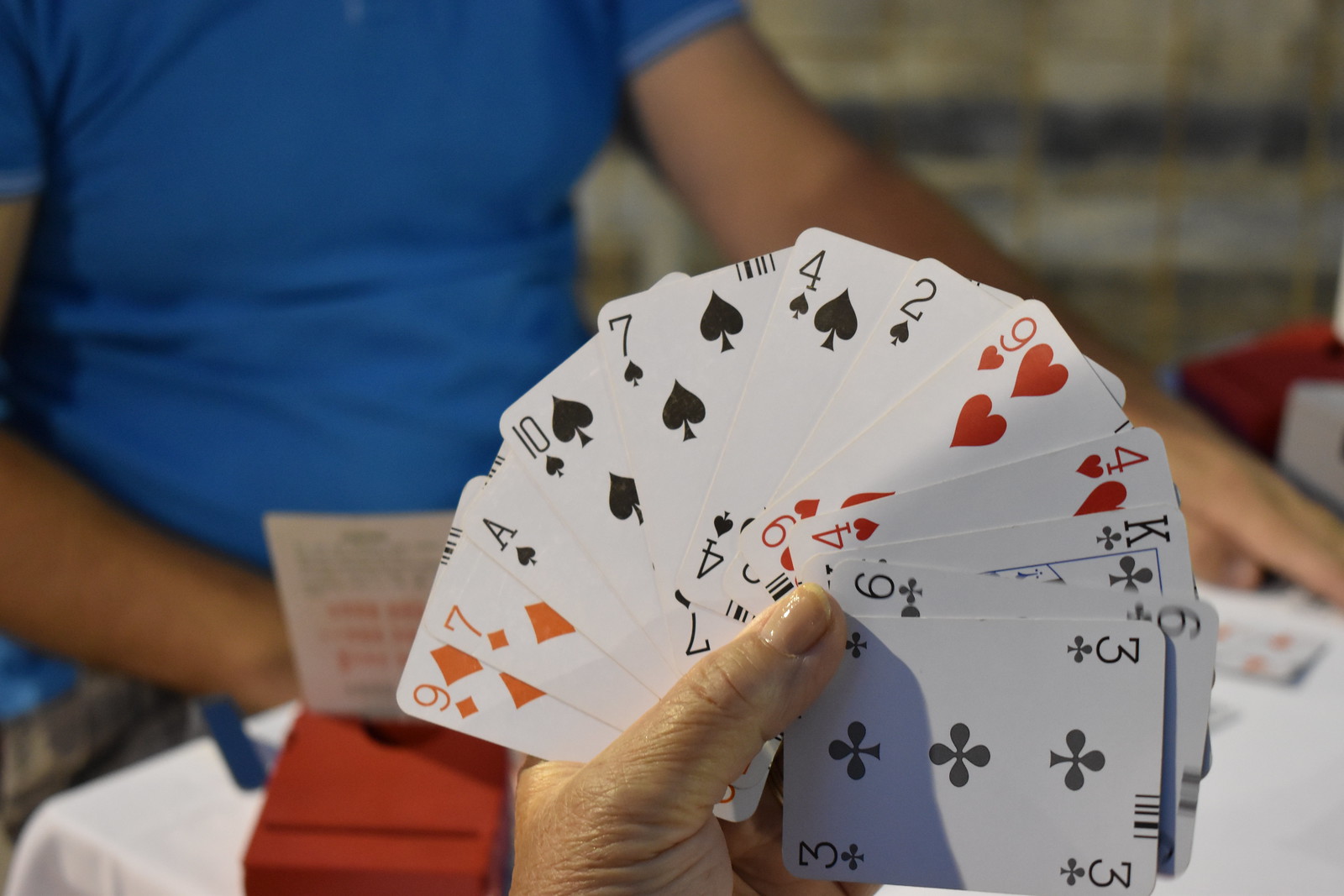In this vibrant color image, a single thumb is visible, holding a fan of approximately a dozen playing cards arrayed in a semi-circular spread, reminiscent of a card player's hand. The cards are facing the viewer, showcasing a variety including the nine of diamonds, seven of diamonds, ten of clubs, king of clubs, and three of clubs. The background features a small table covered with a white tablecloth. Seated at this table is a white individual dressed in a blue short-sleeve shirt, with their left hand resting on the table. This hand is not holding any cards, but there is a single card lying face-up nearby on the right side. The scene is slightly out of focus except for the prominently displayed cards. A red plastic box, typically used for dealing cards, is also present on the table.